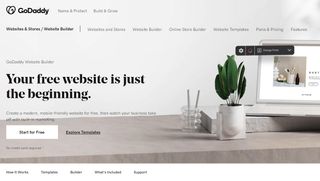A GoDaddy website homepage is displayed, featuring a compact, visually-striking layout. Dominating the page is a large, immersive image of a contemporary desk setup. Central to the desk is a computer monitor, accompanied by a stylish house plant, a ceramic mug, and various artsy decorations, creating a vibrant and modern workspace. 

In the upper left corner, the GoDaddy logo is prominently placed, potentially resembling a butterfly. Overlaying the background image is the slogan, "Your free website is just the beginning," hinting at the platform's broader offerings.

Despite the engaging visual elements, most of the text is too small to be legible. The background reveals an off-white wall, adding to the clean and minimalist aesthetic. Below the banner, a series of links provide navigation options, while additional support and informational links populate the page's footer.

Interestingly, the computer monitor in the main image showcases another meta image: a similar workspace environment featuring a mug filled with pens and pencils, reinforcing the theme of creative productivity.